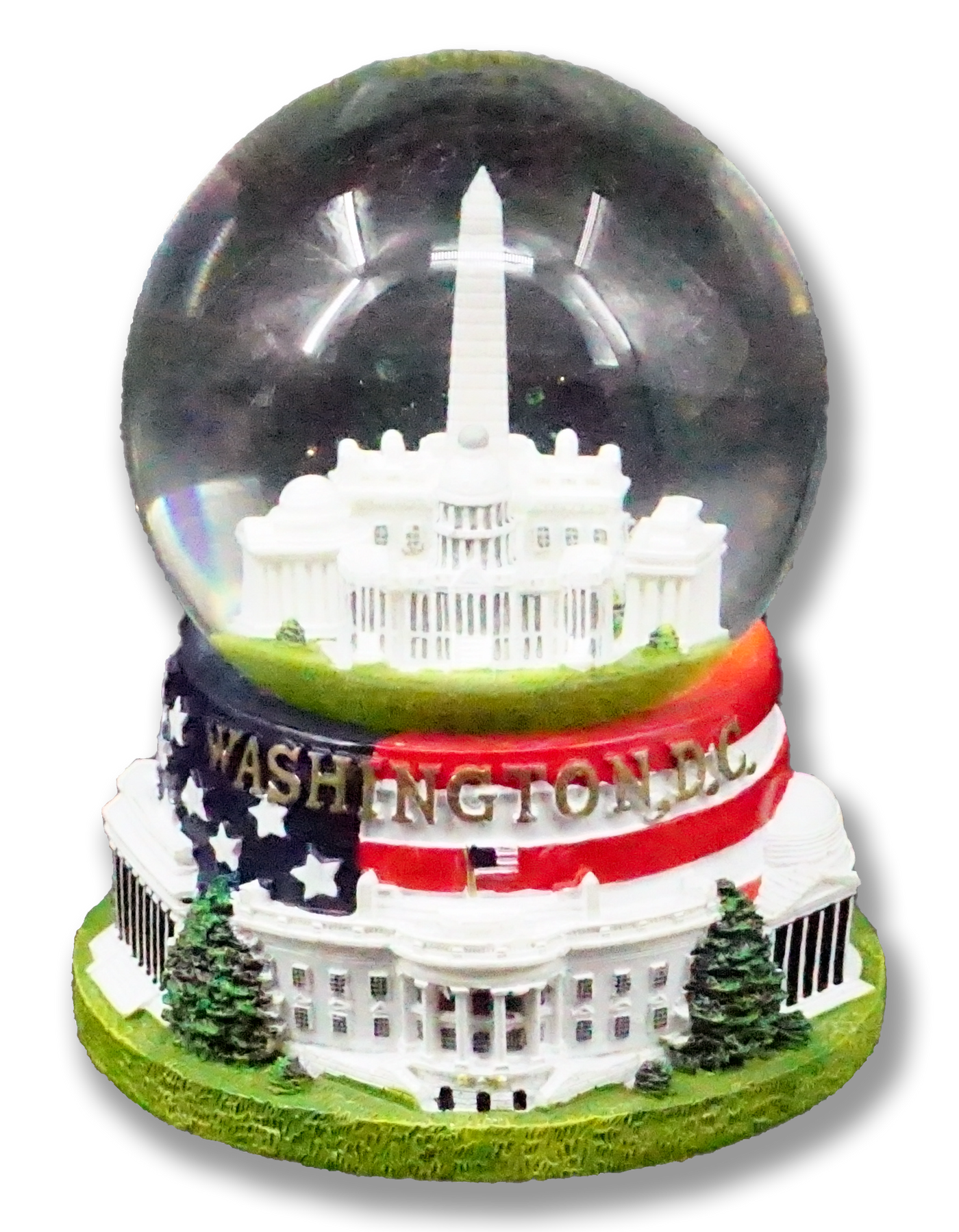The image presents a detailed, close-up view of a Washington, D.C.-themed snow globe. Inside the crystal-clear globe, a model of the White House stands prominently, painted white and accompanied by a small American flag on top. Surrounding the White House, the lush green grass and towering, Christmas tree-like trees create a picturesque scene. Encircling this centerpiece, other iconic landmarks of Washington, D.C., such as the Capitol, the Washington Monument, and the Lincoln Memorial, are visible, adding depth and historical context to the display. At the base of the globe, the words "Washington, D.C." are inscribed in gold over a partial representation of the American flag, symbolizing the patriotic essence of the city. The clarity and brightness of the image, accentuated by the natural lighting, bring out the vibrant colors and intricate details of the snow globe.